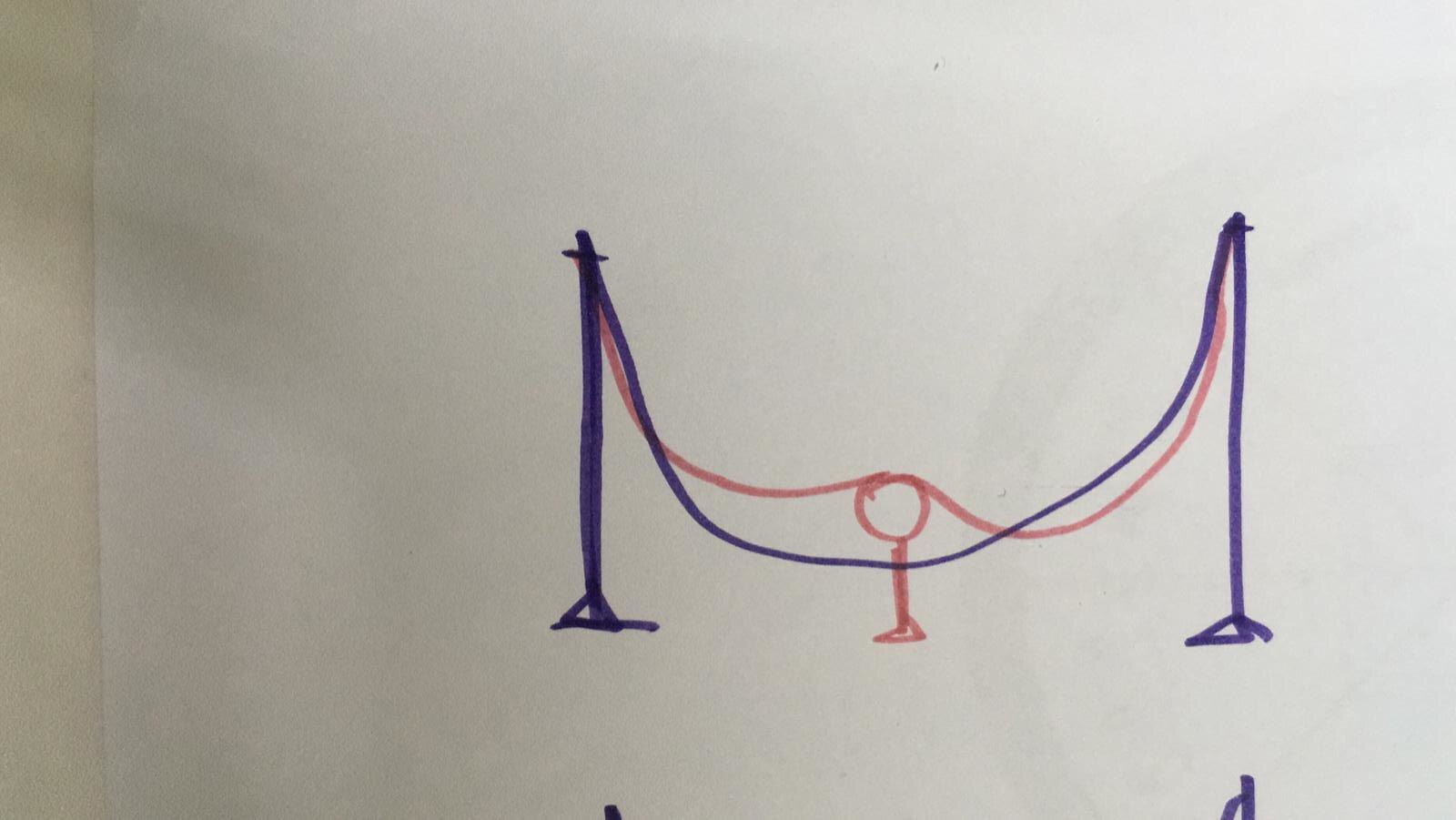A child’s vibrant drawing is centered on a white sheet of paper, placed neatly on another white table. The scene is brightly illuminated, combining both natural and artificial light, casting a soft glow over the entire setup. The drawing itself appears to showcase a whimsical interpretation of a jump rope scene, complete with imaginative elements. 

Two triangle bases anchor poles on either side, connected by a U-shaped line suggesting a rope suspended in mid-air. Alongside this, a pink illustration intersects with a circle, line, and another triangle, possibly depicting a person mid-jump, though its abstract nature leaves room for interpretation. Below the primary drawing, a partial reattempt is visible, with the beginnings of the poles indicated by purple marks.

The artwork is sketched on the reverse side of a document, identifiable by a bold black circle on the right margin, hinting at its original use, perhaps for homework or another formal paper. The combination of childlike creativity and the subtle shadow of its purpose adds an extra layer of charm to the composition.